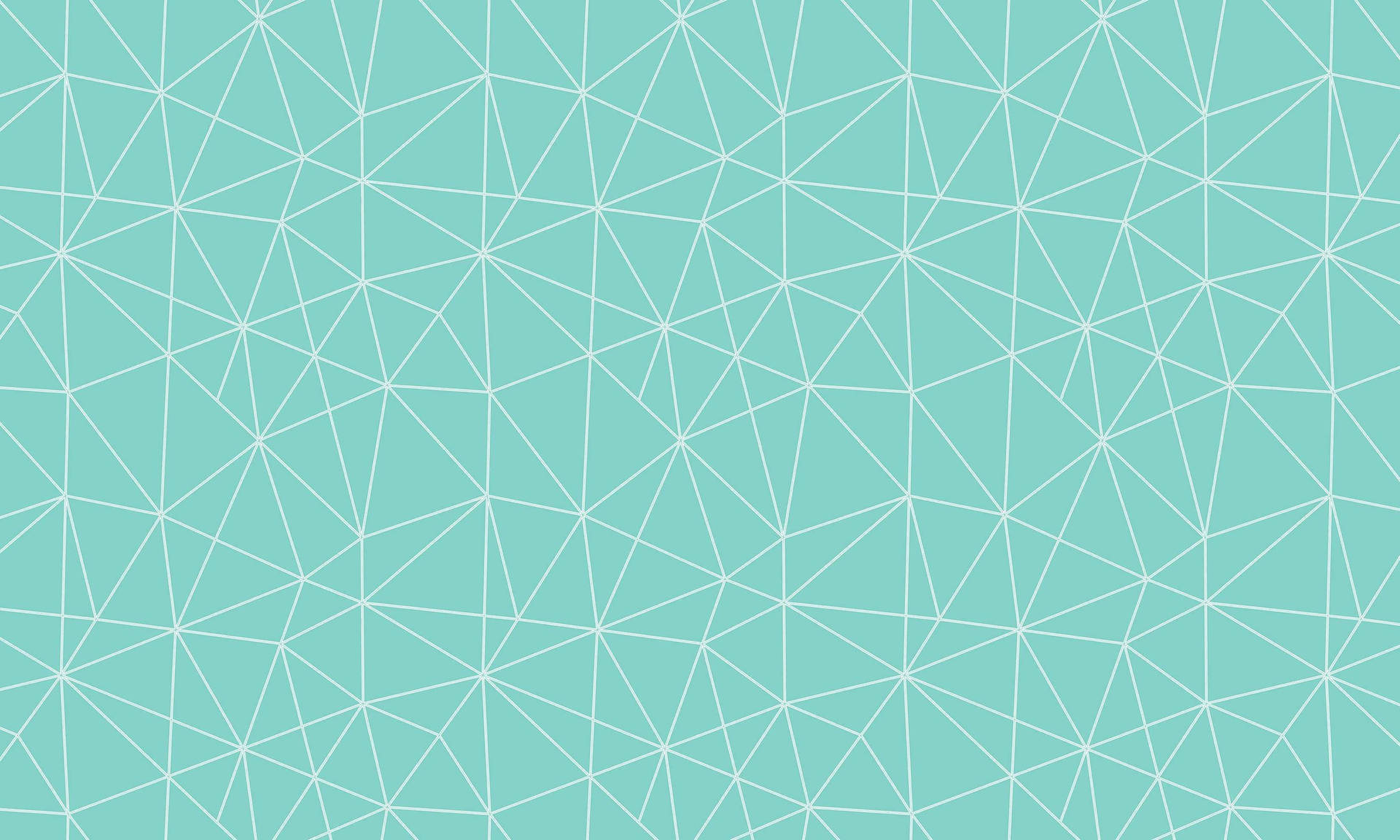This picture is a horizontally presented graphic design featuring a pale aqua blue background with a repeating pattern of delicate white lines. These lines intersect and connect to form a complex array of geometric shapes, predominantly triangles, which sometimes give the illusion of stars, snowflakes, and other polygonal shapes like pentagons and hexagons. The thin white lines create a mesh-like design, giving the entire image a spiderweb-like and abstract appearance. The intersections of the lines form tiny circles or dots, adding a sparkling effect to the overall visual. The pattern is reminiscent of a default computer wallpaper, simple yet intricate, with a consistent repetition of triangles that weave through the entire rectangular image.